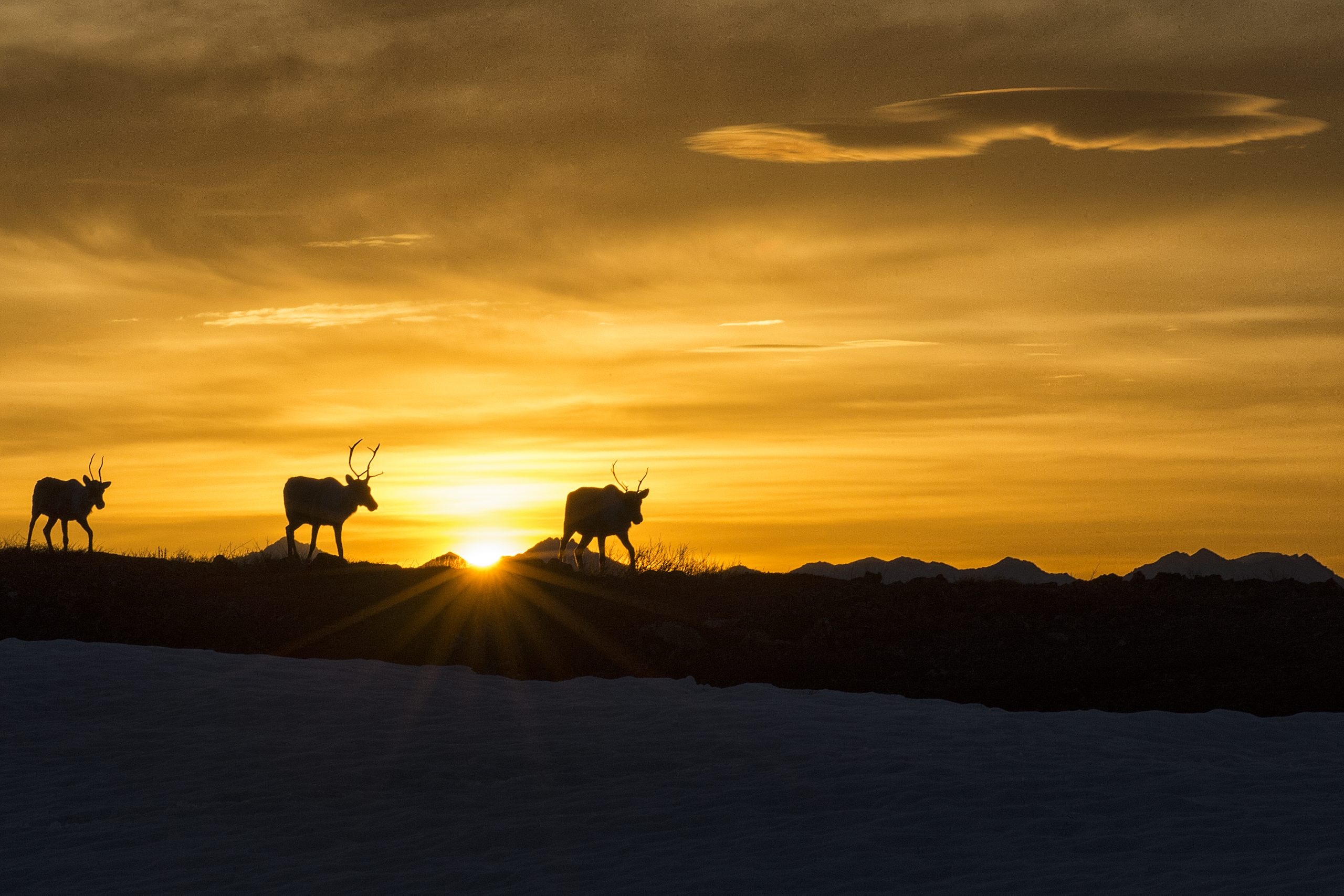In this vibrant and captivating sunset scene, three horned animals, possibly deer, stand silhouetted against a richly hued orange sky streaked with striated clouds. The sun, positioned setting between two of the animals, creates a striking sunburst effect that accentuates their dark shapes. The third animal is positioned far to the left. The creatures are spread out on what appears to be a ridged, rocky terrain at the bottom of the image, bathed in the golden light of the setting sun. The foreground is dark, emphasizing the contrast with the much lighter, almost snowy terrain below. Each animal is distinct in silhouette, with varied antler sizes; the middle animal has notably larger antlers compared to the others. Behind them, the sky dominates the top two-thirds of the photo, with lush colors that suggest both a sense of serenity and the dramatic beauty of nature at dusk.